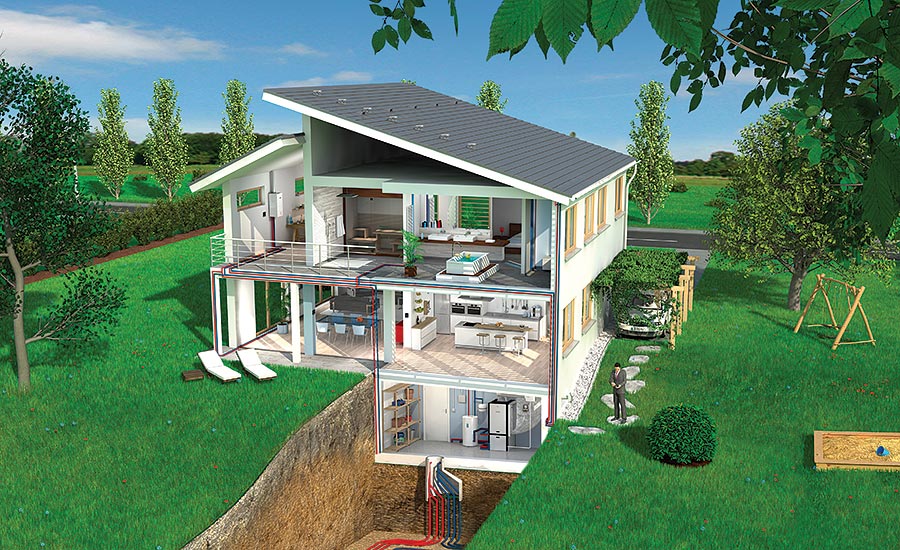This is a highly detailed computer-generated cross-section of a modern, multi-story house, showcasing a well-manicured green yard with various elements like fake trees, a swing set, a sandbox, shrubs, and a stone walkway. The front wall of the house has been sliced off, revealing an interior layout complete with intricate features. The basement, dug into the ground, exposes the piping and wiring systems, along with a hot water heater, furnace, fridge, and shelving units.

On the ground level, the kitchen is depicted with white cabinets and a centrally located island, giving it a contemporary touch. Adjacent is a dining room featuring a blue table and three chairs. The upper level includes a deluxe bathroom with twin sinks and a hot tub, and what appears to be a bedroom or another room, possibly an office. A section of the house has large windows adorned with yellowish trim, providing ample natural light.

The house, painted primarily white with some green and blue beams, features a gray angled roof. In the yard, a person stands, adding a human element to the otherwise artificial scene. Surrounding the house are additional details like a car in a covered carport and a road visible in the background. The blue sky with several clouds suggests a pleasant daytime setting.